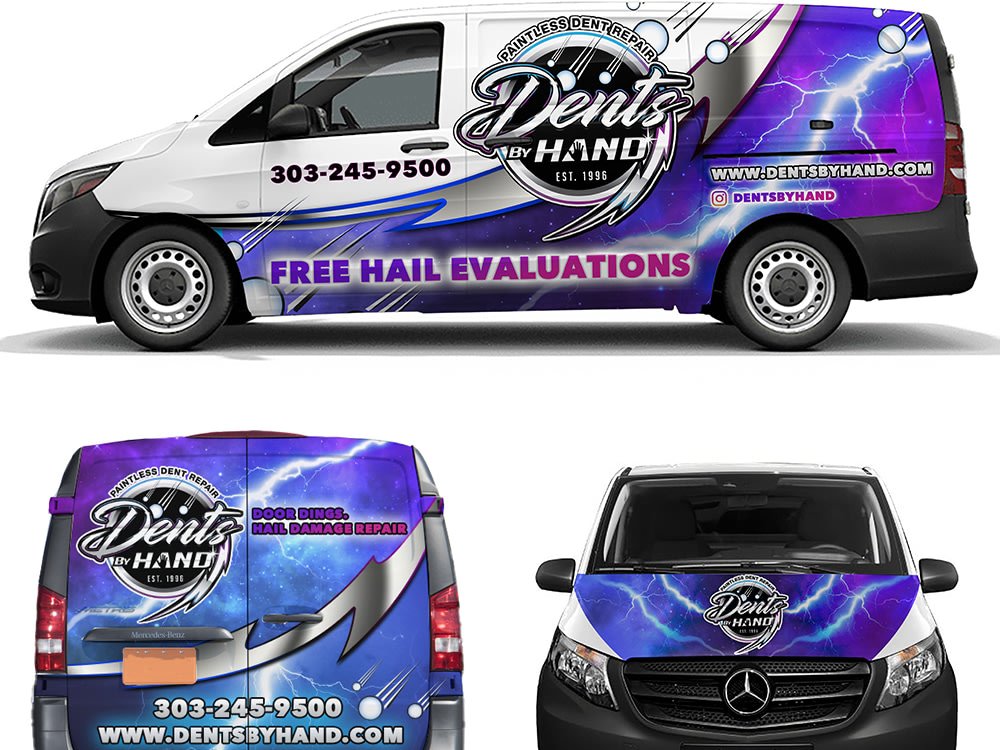**Advertisement for Dents by Hand: Three-View Photograph Collage of Branded Mercedes Van**

This advertisement showcases a tri-view collage of a branded Mercedes van for Dents by Hand, an established business specializing in paintless dent repairs since 1996. The van itself is a newer model, prominently painted in white with accents of purple and black.

1. **Side View**: The left side of the van is highlighted at the top of the collage. Here, the main branding is displayed in a circle decal, reading "Dents by Hand, Paintless Dent Repair," and it proudly states "Established 1996." Below, near the rocker panel, it offers "Free Hail Evaluations." Noteworthy is a silver lightning bolt graphic running horizontally across the side of the van.

2. **Back View**: Located in the lower left corner of the collage, the back of the van mirrors the information on the side. "Dents by Hand" is prominently displayed on the left door. At the bottom of both doors, the contact details are provided: a phone number (303-245-9500) and the website "www.dentsbyhand.com."

3. **Front View**: The front of the van, shown in the right corner of the image, features the signature Mercedes emblem on the grill. Additionally, the logo "Dents by Hand" is visible on the hood against a blue background.

Across all views, social media information is also visible, with an Instagram handle (@dentsbyhand). This detailed visualization effectively communicates the comprehensive branding and contact information of Dents by Hand, emphasizing their expertise in dent repair services.